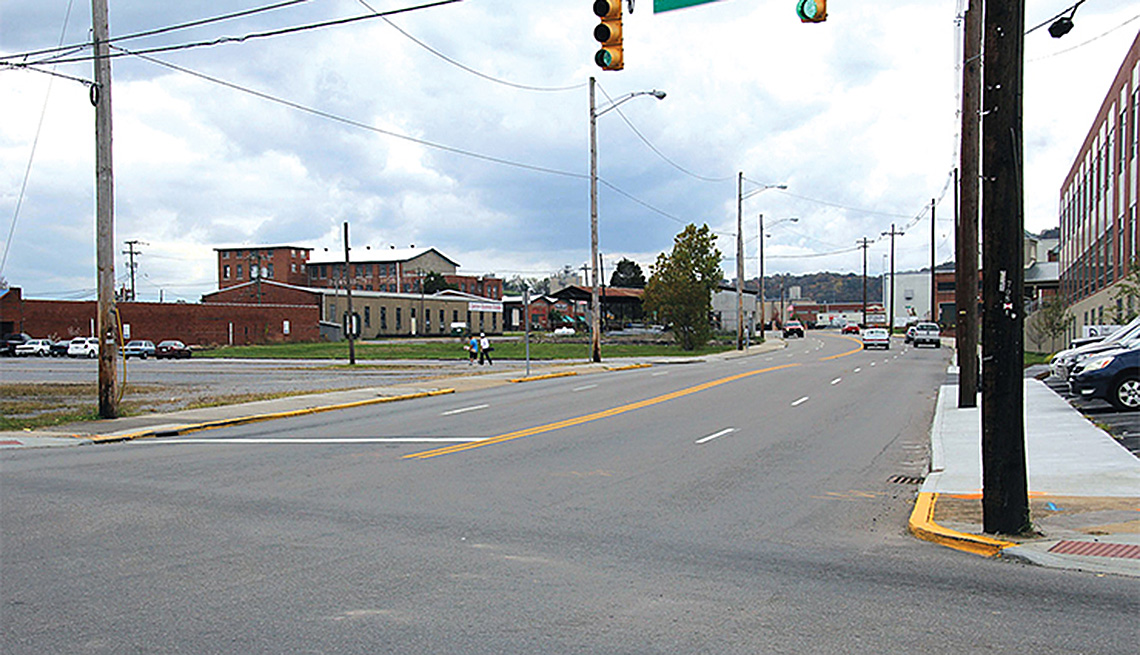This is a daytime photograph of a city street captured in a horizontal rectangular frame. The sky above is light blue with a significant cover of light gray, puffy clouds. The wide, four-lane paved road stretches down the center, divided neatly into two lanes in each direction by a solid yellow stripe with white dashed lines on either side. Several cars are visible, some heading towards the camera on the left side and others driving away on the right.

On the right side of the street, there is a white sidewalk equipped with tall, black poles and what appears to be a parking area extending further along. The left side of the street also features a sidewalk where a few pedestrians can be spotted in the distance. This side is lined with buildings, a few of which have light brown and dark red facades. Additional buildings with varied architectural styles, including some multi-storied ones and houses with triangular roofs, form the background.

There is a streetlight positioned centrally in the image showing a green light, indicating that vehicles are allowed to proceed. Besides the streetlights, numerous lampposts and electrical poles are scattered throughout the scene, enhancing the city's infrastructure.